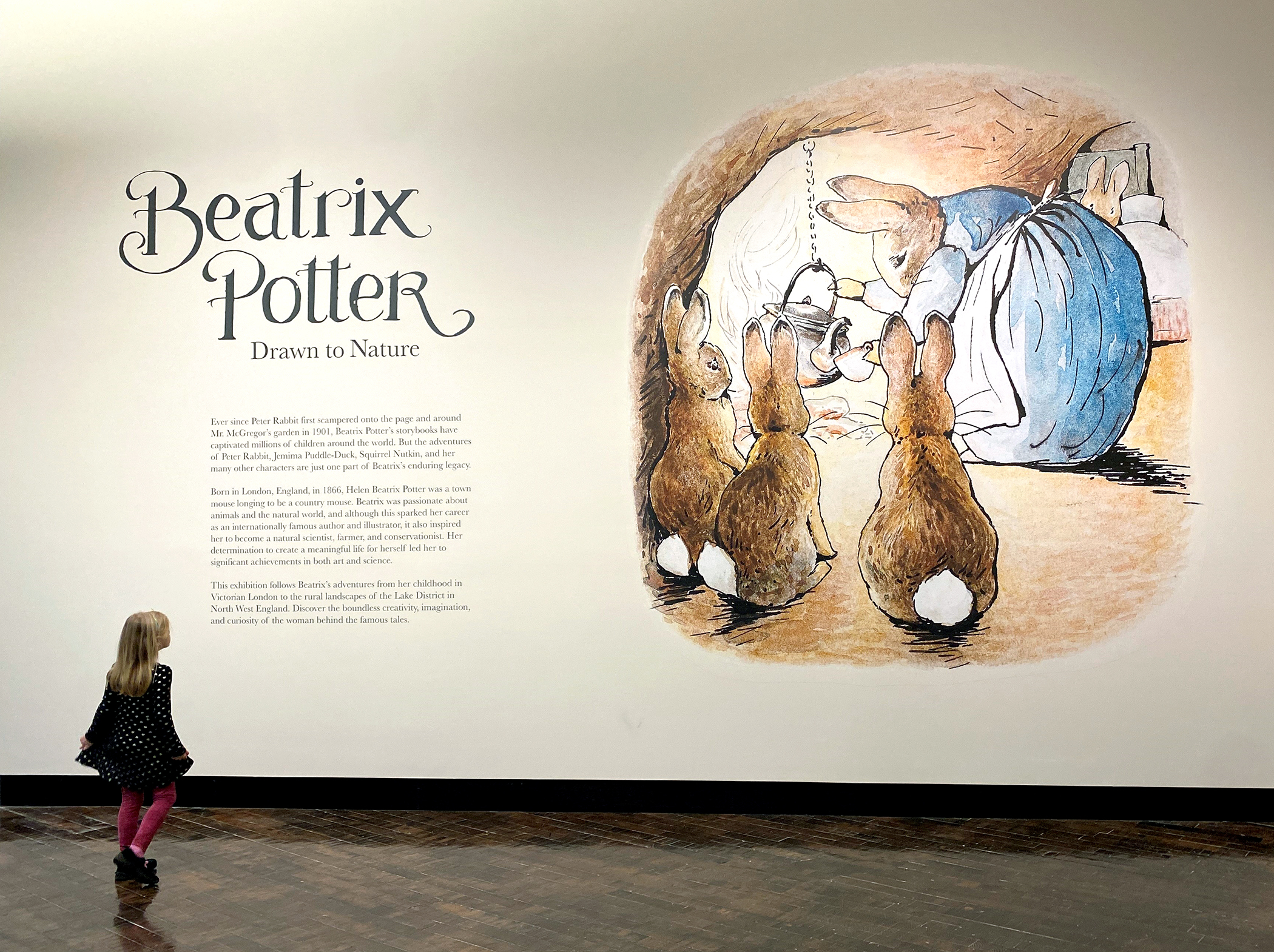In an indoor setting, a small girl, seen from the back, is seated on the floor, intently gazing at a large poster mounted on the wall. She is dressed in a black dress adorned with white polka dots and wears pink tights. The poster, titled "Beatrix Potter: Drawn to Nature" in large letters on the left side, has a white background with black text detailing the life and works of Beatrix Potter. Illustrations on the poster depict a scene with anthropomorphic rabbits: a large rabbit in a blue dress is pouring tea from a teapot that hangs over a fire in what looks like a cave setting. Nearby, three smaller rabbits watch attentively, while another rabbit is seen in the background lying in a bed. The text recounts Beatrix Potter's passion for the natural world, her journey from Victorian London to the rural Lake District, and her legacy as an author, illustrator, natural scientist, and conservationist.